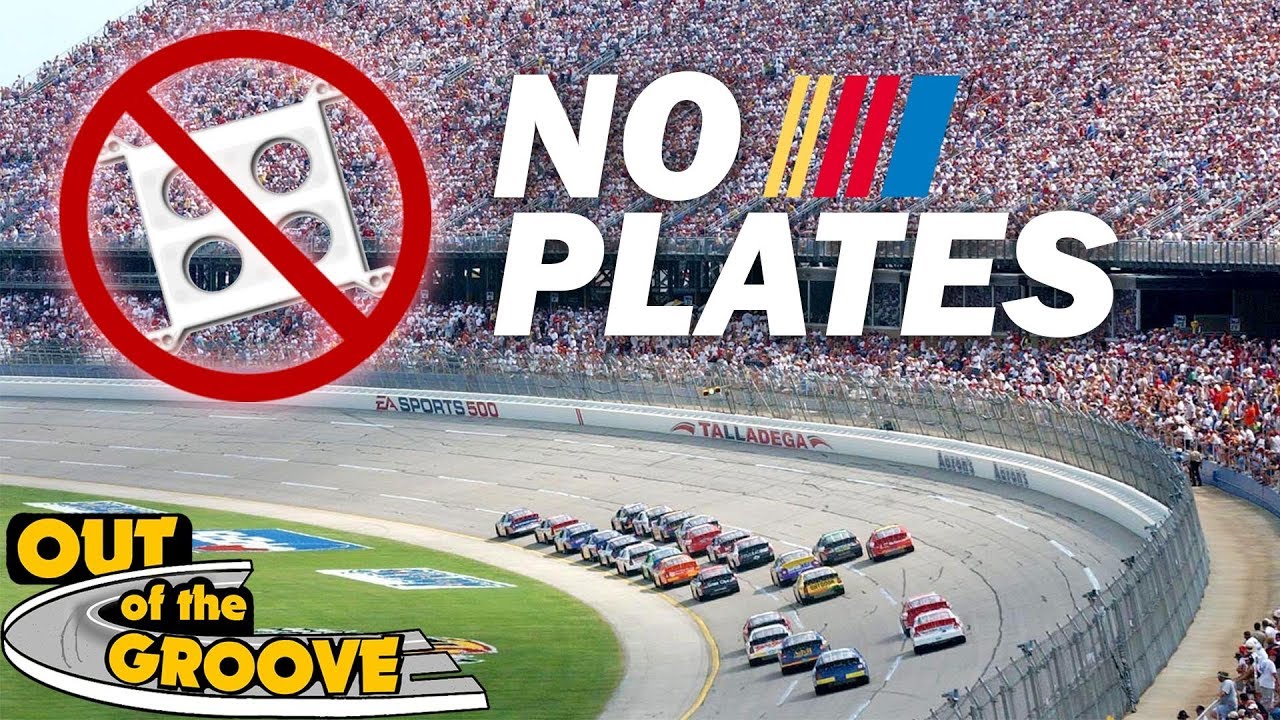The image depicts a bustling racetrack stadium, packed to capacity with thousands of spectators. The stadium, expansive and curved, wraps around a racing strip where about 20 cars are seen competing, arranged in two pace lines. The viewpoint is slightly elevated, allowing a clear view of the stadium’s structure and the lively crowd in the stands. Dominating the background are advertisements: "EA Sports 500" is emblazoned across the racetrack wall, followed by the name "Talladega" in bold red and black letters. Above this, a sign reads "no plates" with an illustrative graphic—a square with four circles inside, crossed out with a red slash, indicating a prohibition. The bottom left corner features the phrase "out of the groove" in yellow letters. A tall fence secures the perimeter of the racetrack, and a patch of greenery is vaguely visible to the left. The scene is set on a bright, sunny day, amplifying the excitement and energy of the racing event.